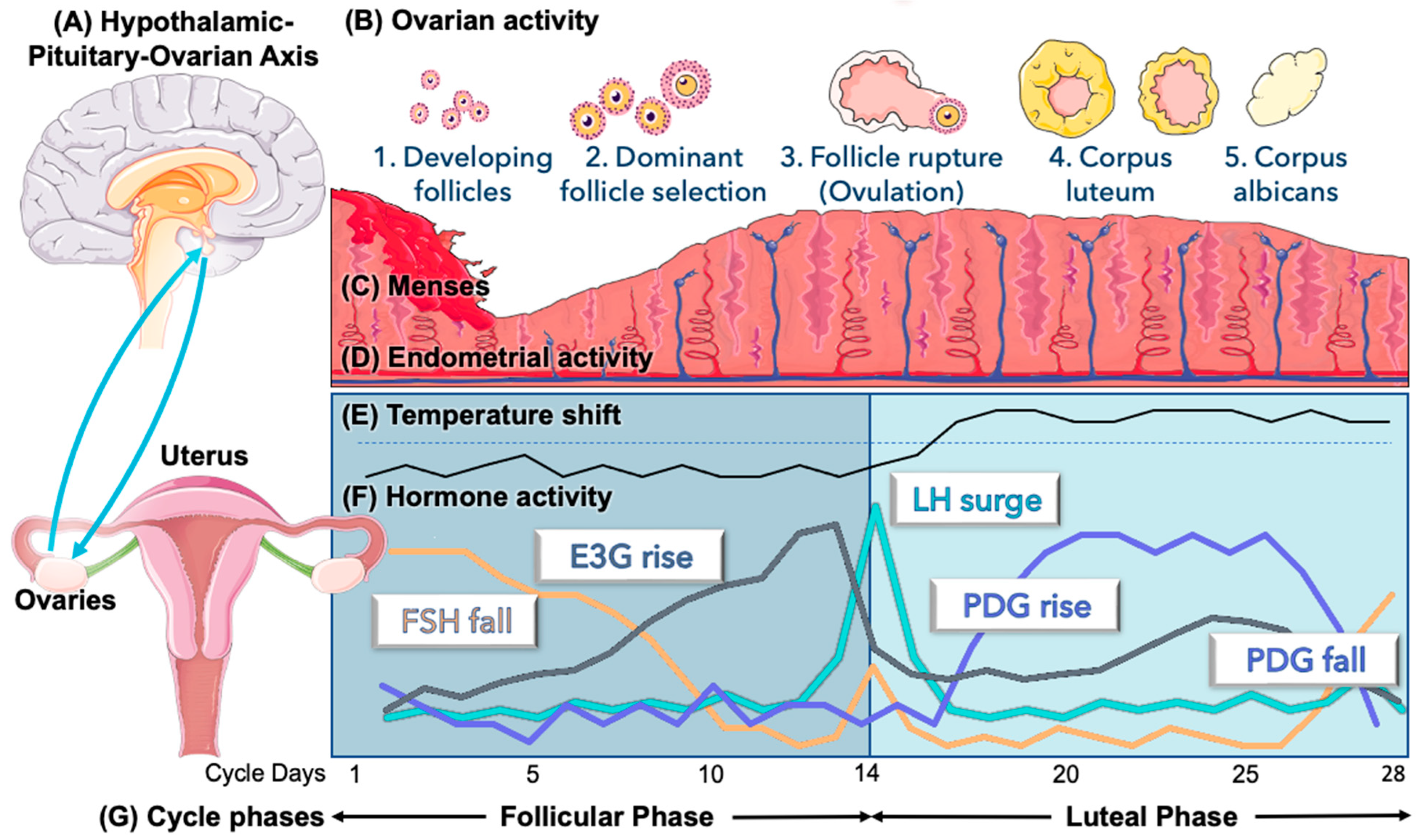The image is a detailed medical diagram illustrating the female reproductive system and its associated hormonal cycles. In the upper left corner, labeled "A," is a purple drawing of the hypothalamic-pituitary-ovarian axis, showing connections between the brain and the ovaries via blue arrows pointing to a light cream-colored bulb labeled "ovaries" and "uterus." Above this, the black text reads "hypothalamic-pituitary-ovarian axis."

To the right, section "B" focuses on ovarian activities, with five bullet points detailing the stages: 1. Developing follicles, 2. Dominant follicle selection, 3. Follicle rupture, 4. Corpus luteum, 5. Corpus albicans. Below this is a red, pink, and purple graph, labeled "C" (mensis) and "D" (endometrial activity), with blue lines pointing upwards.

Further down, section "E" describes temperature shifts, while section "F" illustrates hormone activity with a graph showcasing various colored lines (black, yellow, gray, teal, blue, orange) labeled with FSH fall, E3G rise, LH surge, PDG rise, PDG fall, and cycle days 1, 5, 10, 14, 20, 25, and 28. The bottom-most part, labeled "G," indicates the cycle phases: follicular phase and luteal phase, separated by black lines with points marking different stages.